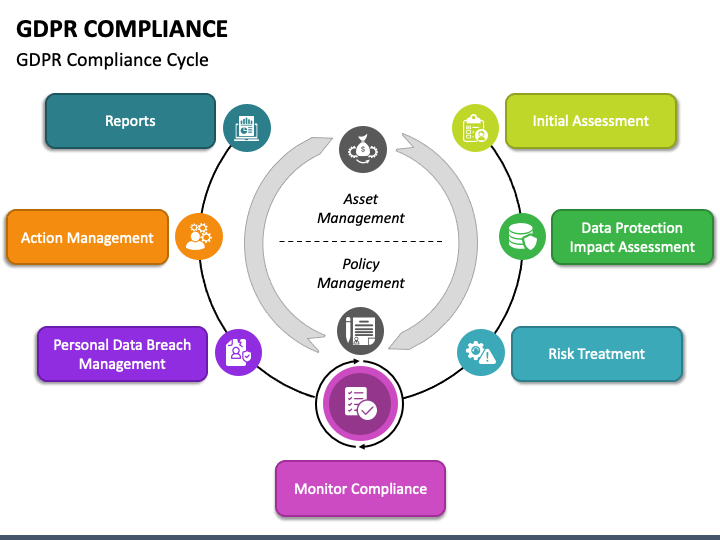The image is a detailed PowerPoint presentation slide with a white background and a black border at the bottom. The top left corner prominently features the bold black heading "GDPR Compliance," followed by the subtitle "GDPR Compliance Cycle." Centrally, a cyclical or circular design is displayed, encircled by various colored rectangles and circles representing different stages of the GDPR compliance process.

The central circle highlights "Asset Management" on top, underlined by a dotted line, and "Policy Management" below it. Each of these is accompanied by a grey circular icon: a coin bag with a dollar sign for Asset Management and a pen and paper for Policy Management. Surrounding this central circle is a grey ribbon-like ring, bordered by a black circular ring displaying additional icons in various colors.

Starting from the top-right and moving clockwise, the stages include:
1. "Initial Assessments" in a lemon-colored rectangle with a green clipboard and face icon.
2. "Data Protection Impact Assessment" in a dark green rectangle with a shield and circular objects icon.
3. "Risk Treatment" in a light blue rectangle featuring a settings icon and a danger sign.
4. "Monitor Compliance" in a pink rectangle with a notepad sporting tick marks and lines icon.
5. "Personal Data Breach" in a purple rectangle with an icon of a page, human figure, and shield with a tick sign.
6. "Action Management" in an orange rectangle with a human figure and three settings button icon.
7. "Reports" in a dark green rectangle with an icon of a box or computer screen with papers behind it.

These phases collectively form an almost complete circle, visually representing the continuous process cycle of GDPR compliance.